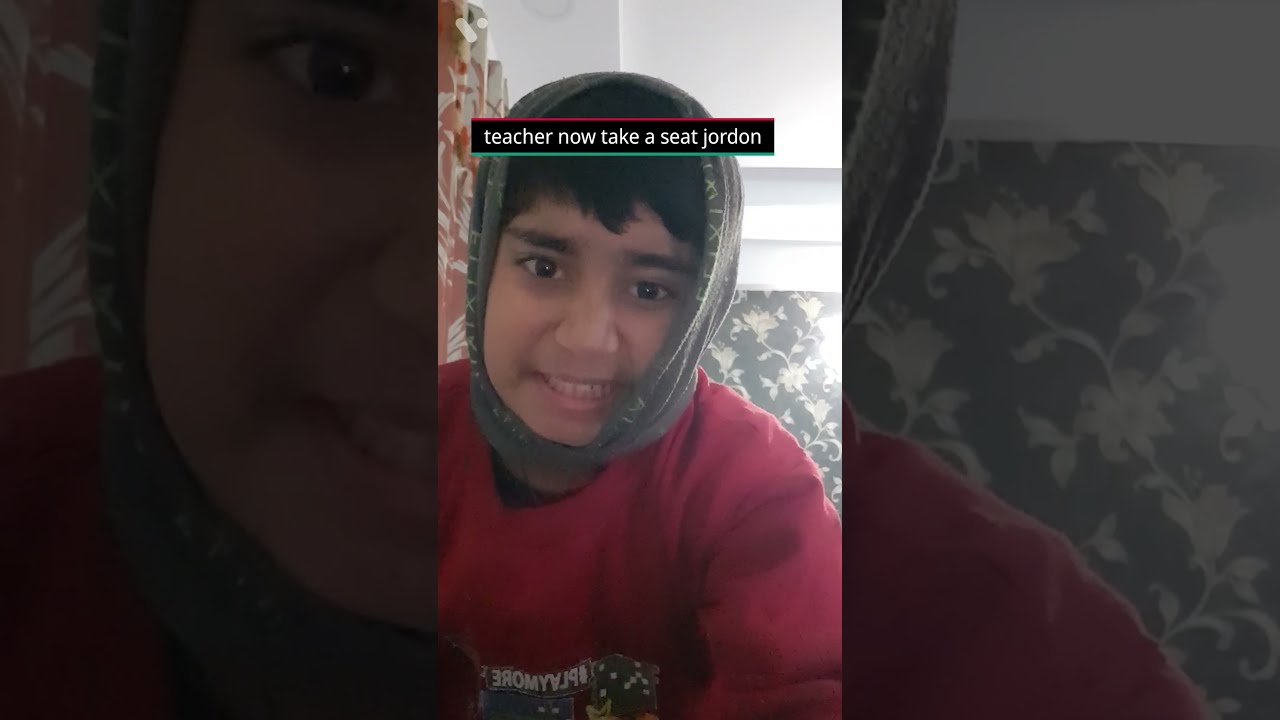The image is a screen grab from a video taken in a smartphone aspect ratio, featuring a teenager of undetermined gender with light brown skin and black hair. The young person, possibly around 14 or 15 years old, wears a gray headscarf and a red long-sleeve shirt over a black undershirt. They are seated on a couch with a flowery wallpaper and a white window in the background. The scene is likely from a personal video or a video chat, and the expression on the teenager's face is a mix of apprehension and focus, with their mouth slightly open and teeth gritted. A black banner with a red and green border appears at the top of the screen, bearing the caption, "Teacher now take a seat Jordan," suggesting a classroom setting. The photograph has been edited to be darker and enlarged at the sides, adding depth to the composition.